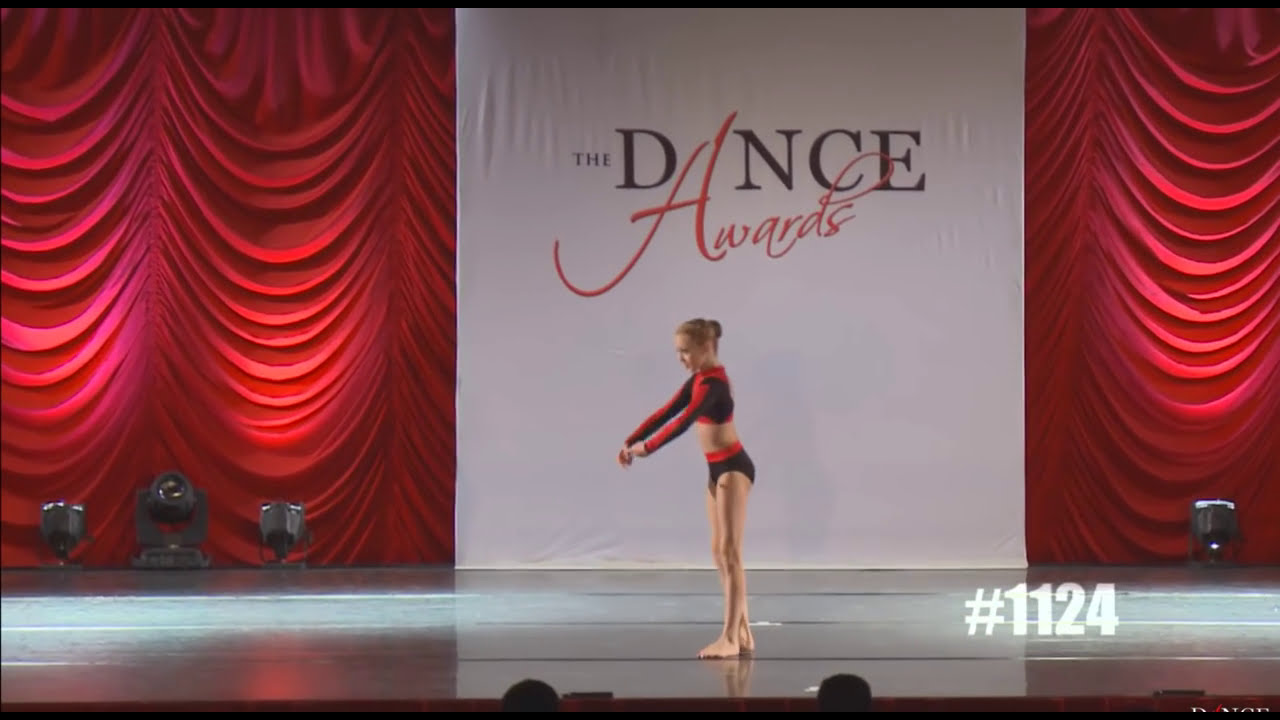In the image, a young girl with light brown hair, dressed in a black and red dance outfit that exposes her midriff, stands in a graceful dance pose on a metallic-gray stage, which is well-lit. She is wearing a red and black long-sleeve top and matching bikini-style bottoms. The stage is set with rose-colored, fancy red curtains draped across the backdrop. Prominently displayed near the center-right is a large white panel with the text "Dance" in bold black letters and "Awards" in matching red font, written in cursive, with the "A" shared between the two words. The number "1124" can be seen in white block letters on the stage. Theater lighting and possibly the beginning of an audience are visible at the bottom edge of the image.